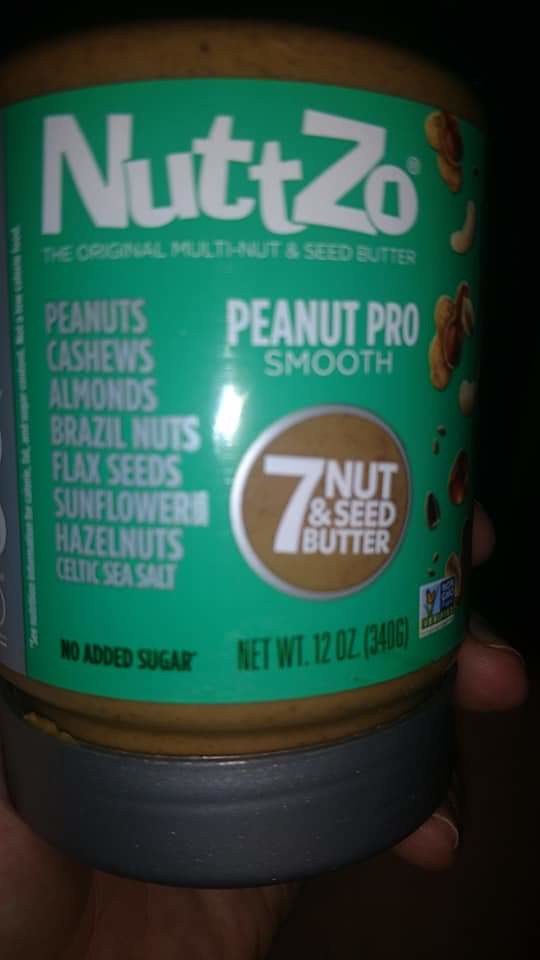The photograph captures an indoor setting where an individual is holding up a 12-ounce jar of Nutzo "The Original Multi-Nut and Seed Butter Peanut Pro Smooth". The jar features a green label adorned with white lettering. On the left side of the label, there is a list of ingredients, clearly stating: peanuts, cashews, almonds, Brazil nuts, flaxseed, sunflower seeds, hazelnuts, and Celtic sea salt, with an emphasis on no added sugar. On the right side of the label, there are illustrative pictures of the various nuts and seeds included in the butter, arranged vertically. Prominently displayed in the center of the label is the phrase "Seven Nut and Seed Butter," underscoring the product’s unique blend.